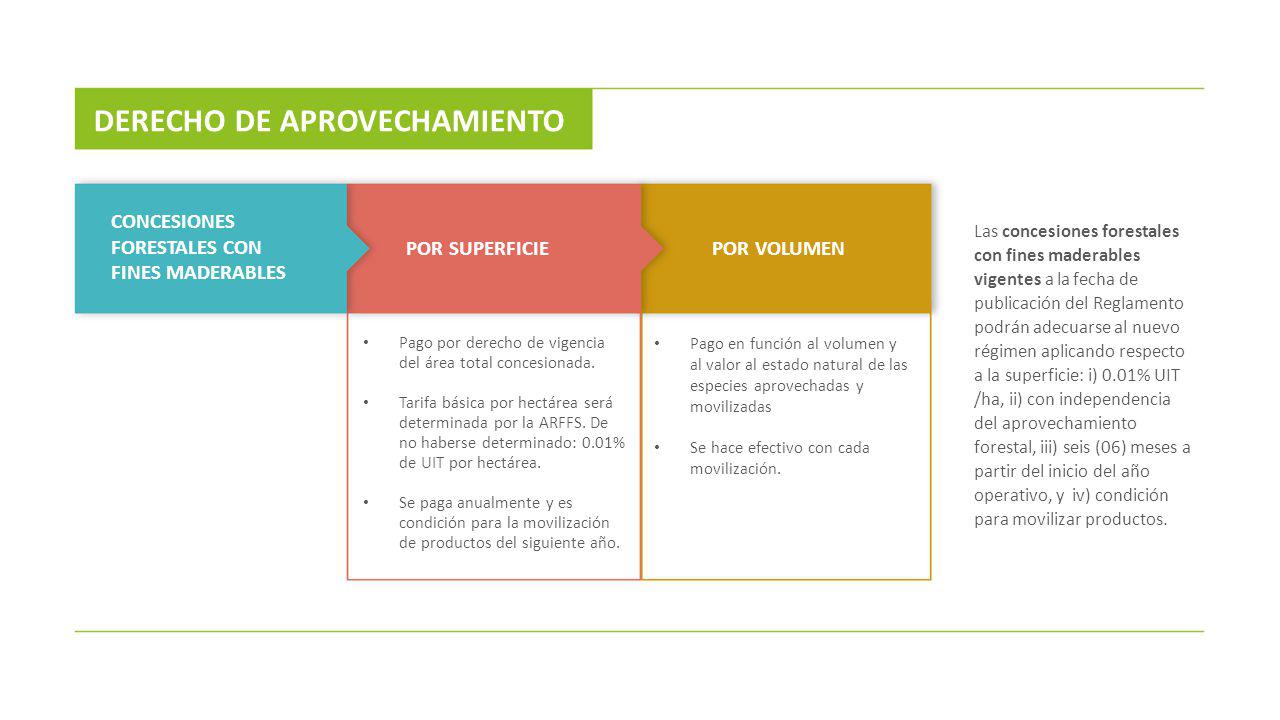The image appears to be a page from a book or document, featuring text mainly in Spanish. It is framed with thin green lines at the top and bottom. On the top left, there's a large green rectangle that contains white text reading "Derecho de aprovechamiento." Directly below this is a blue rectangle with a right-pointing arrow halfway out of its right side, displaying the text "Concesiones forestales con fines moderables" in white font. 

This blue rectangle connects to a red rectangle with the white text "Por superficie," which extends downward and contains a list of items in Spanish, indicated by dots. The red rectangle is followed by an orange rectangle with the text "Por volumen," also featuring additional dots listing more Spanish terms. Adjacent to these boxes, on the far right, there is a paragraph of text all in black font. The interconnected shapes of the rectangles resemble puzzle pieces, but with triangles instead of the typical interlocking circles.